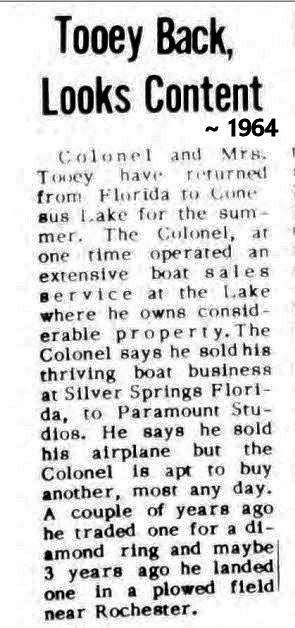This image depicts a screenshot of a small strip from an old newspaper or magazine article with a white background and black text. The title reads "Tooey Back, Looks Content, 1964" in large type. Beneath the title is a vertical column of smaller black text: "Colonel and Mrs. Tooey have returned from Florida to Constance Lake for the summer. The colonel at one time operated an extensive boat sales service at the lake where he owns considerable property. The colonel says he sold his thriving boat business at Silver Springs, Florida, to Paramount Studios. He says he sold his airplane, but the colonel is apt to buy another most any day. A couple of years ago, he traded one for a diamond ring, and maybe three years ago, he landed one in a plowed field near Rochester." The image has a few visual imperfections, such as a black bar at the top, a faint black bar along the right edge, and varying degrees of text blurriness, indicating it is indeed a captured image of an aged print article.